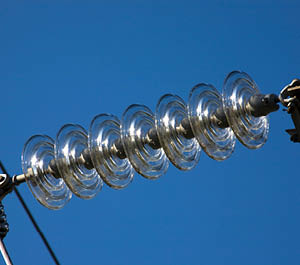The photograph features a dark blue sky as the background with a rod or wire extending diagonally across the middle of the image, tilting upwards to the right. Suspended on this rod are seven clear, round glass discs, each with engraved details including two to three ridges. These discs reflect light at a consistent angle, producing a visible glare. Each disc is spaced by a small gray ball, and both ends of the rod show some mechanical-looking distortions. In the bottom left corner, there is a partially visible white cord or wire, presumed to be electrical, suggesting the setup might be part of an overhead telephone or power line system.